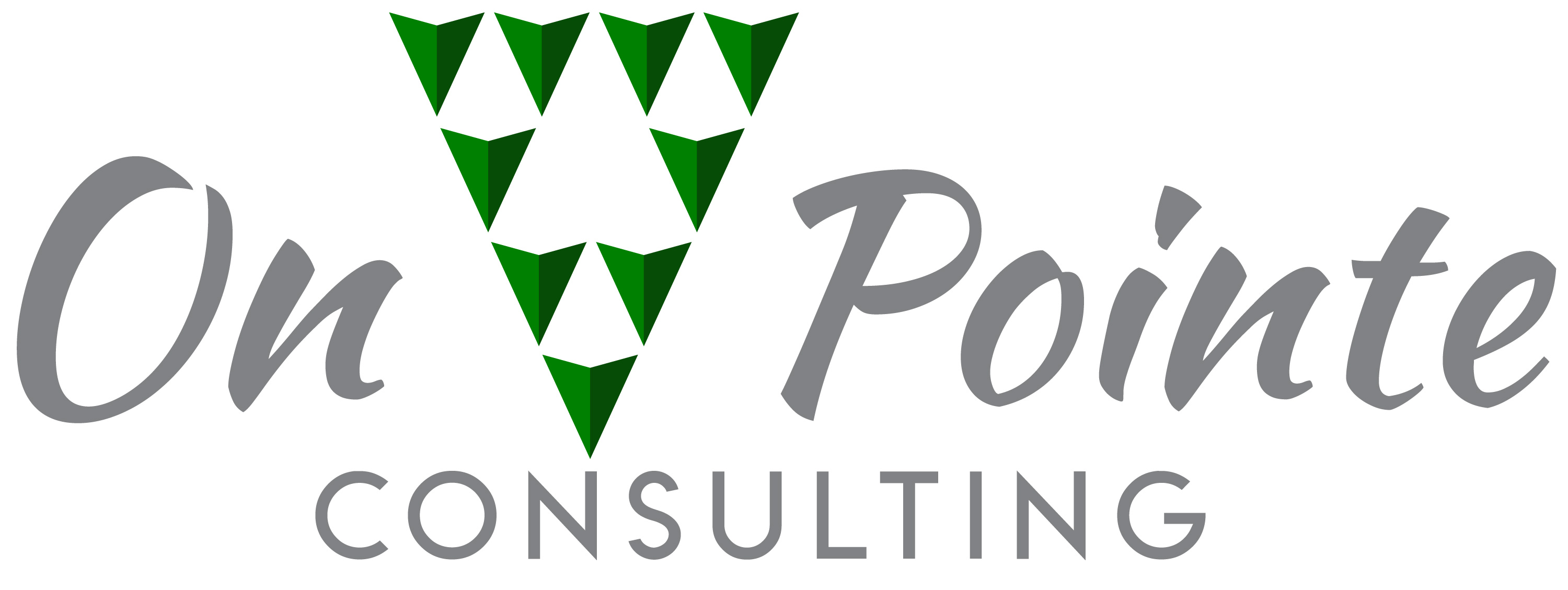The image displays a commercial logo for the company "ON POINT CONSULTING." The logo is set against a white background and features the text "ON POINT" in grey, italicized lettering, with "CONSULTING" written below in uppercase grey block letters. Central to the logo is a distinctive triangular motif comprising smaller green triangles. This main triangle is upside down and depicts a complex Escher-like, geometric pattern. Specifically, it consists of four rows of triangles: the top row has four green triangles, the second row has two triangles separated by a space, the third row has two green triangles, and the bottom row features a single green triangle. The triangles are rendered in shades of light and dark green, creating a dynamic, visually engaging effect. The overall intricate design leaves white triangular spaces that suggest facial features like eyes, a nose, and a mouth, making the logo both memorable and visually striking.